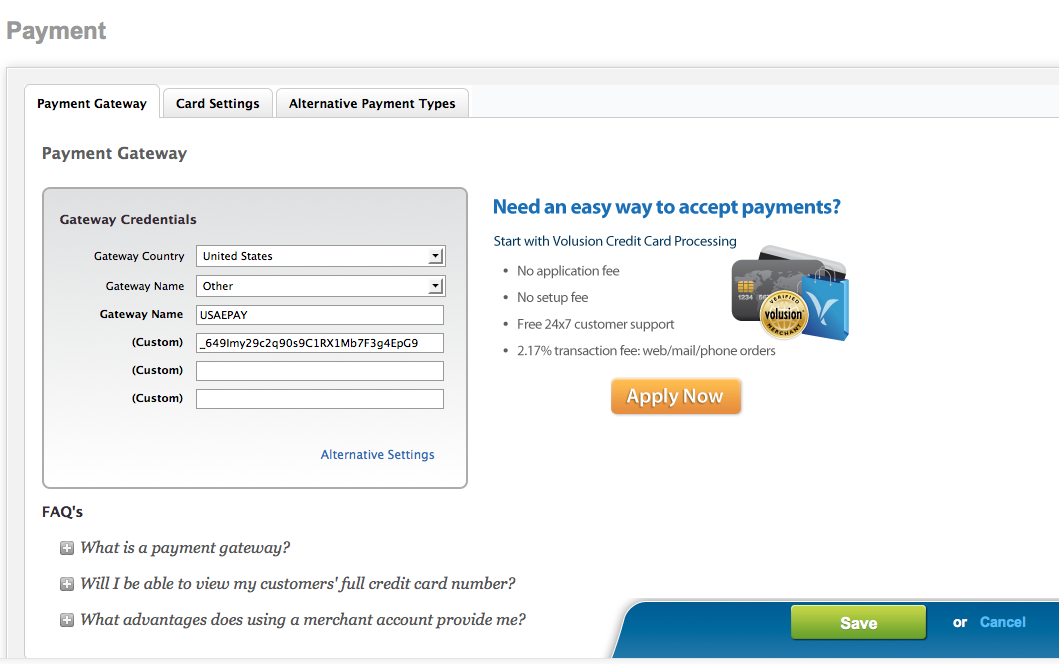The image depicts an outdated-looking payment gateway screen, designed for processing credit card transactions. The interface highlights the ease of accepting payments, prominently featuring benefits such as no application fee, no setup fee, and free customer service. The vintage-style design and simplistic layout offer a nostalgic journey back to earlier days of web aesthetics, underscoring user-friendly features amidst an old-school digital environment.